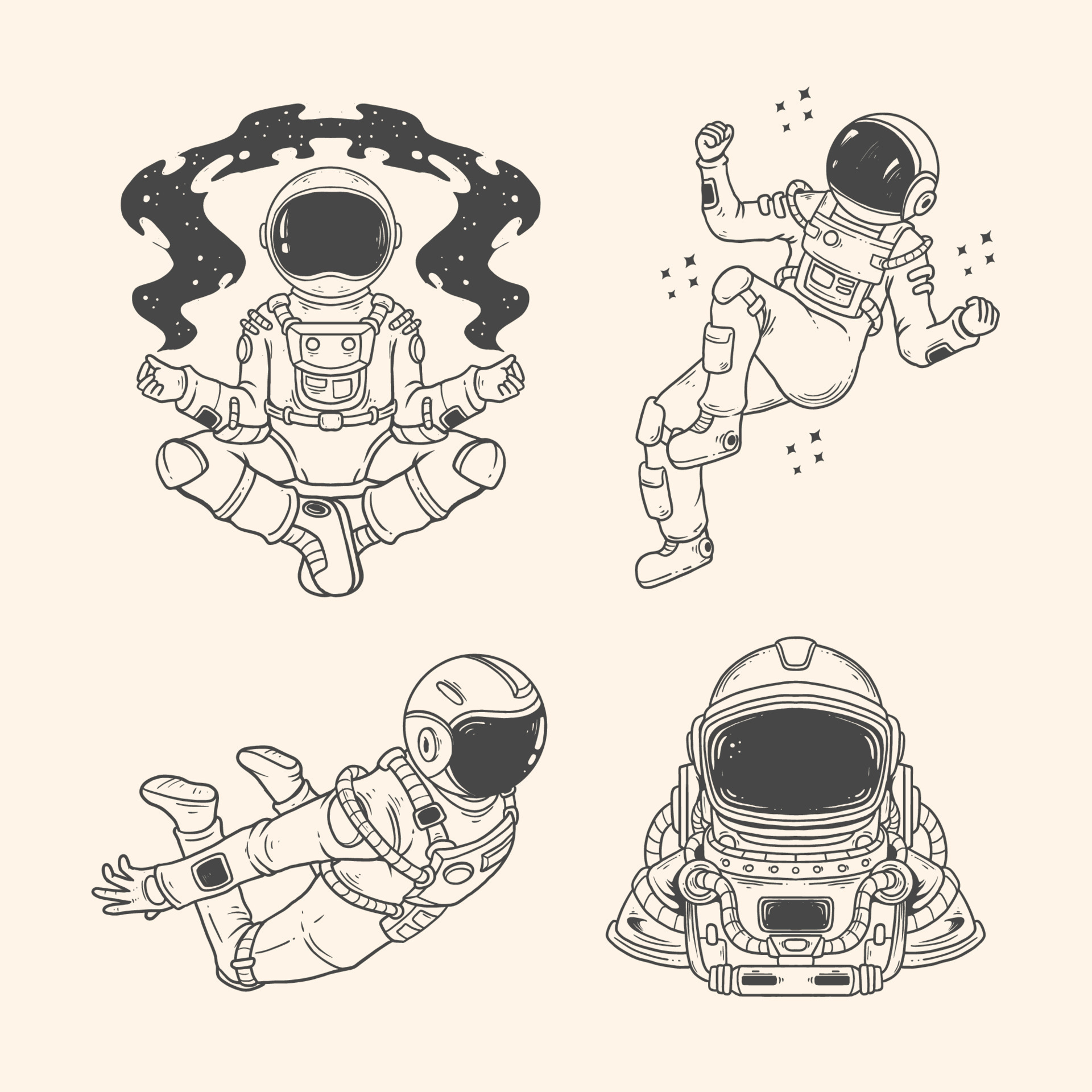This image features four distinct, cartoon-style drawings of astronauts, each positioned in a corner of the frame. The top left shows an astronaut in a spacesuit, sitting cross-legged in a meditation pose, with their hands making a mudra gesture. Above their fingertips, space and stars flow upward, creating a serene cosmic backdrop. The top right corner depicts a fully covered astronaut dancing gracefully in space, surrounded by twinkling stars. The bottom right focuses on a close-up of an astronaut's helmet and shoulders, highlighting the intricate details of the spacesuit gear. Lastly, the bottom left presents the full body of what appears to be the same astronaut, captured in a dynamic pose, as if jumping with bent legs and arms tucked behind, giving an impression of floating effortlessly through space. The images collectively suggest various activities of an astronaut in outer space, rendered with detailed, computer-generated graphics.